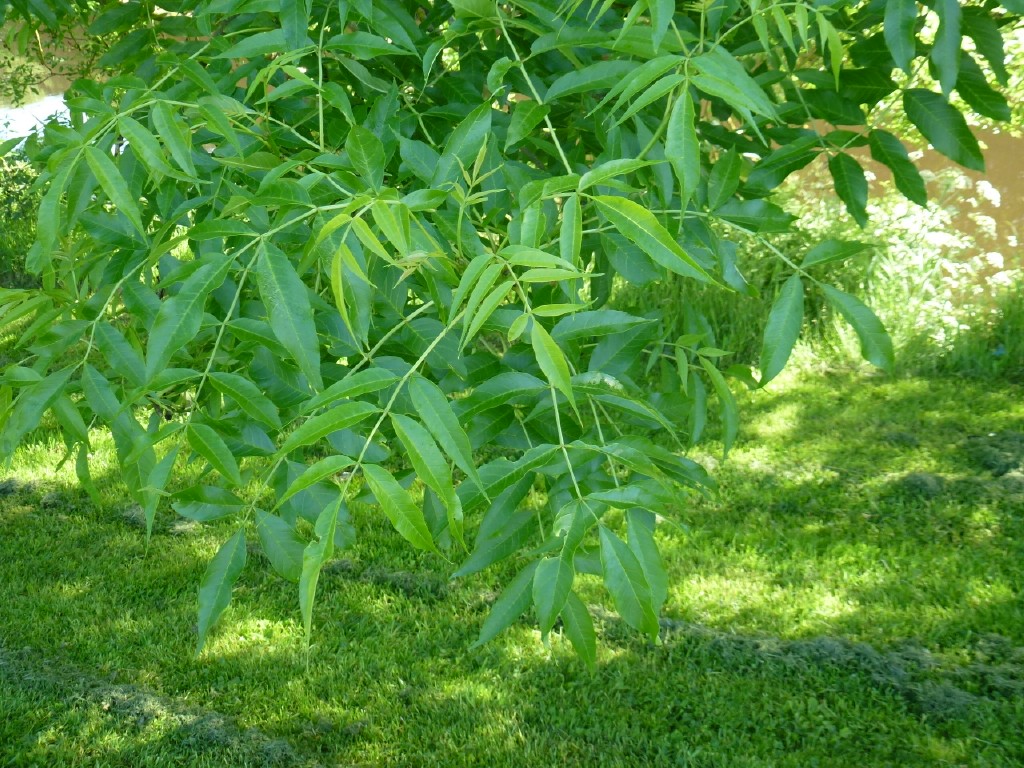The photograph captures an outdoor scene along the bank of a river or pond, featuring freshly mowed grass with scattered grass clippings across the bottom of the image. Dominating the central portion of the photo are the branches of a lush, green bush or tree, densely packed at the top and extending downward and outward toward the left and right sides. In the top left-hand corner, one can discern a bank behind the bush, with hints of water and land on the opposite side. The top right-hand corner reveals some white flowers and brown water, with additional greenery visible beyond. Sunlight pierces through, adding a gentle glow, particularly noticeable in the lower right quadrant where the mowed grass is faintly illuminated.